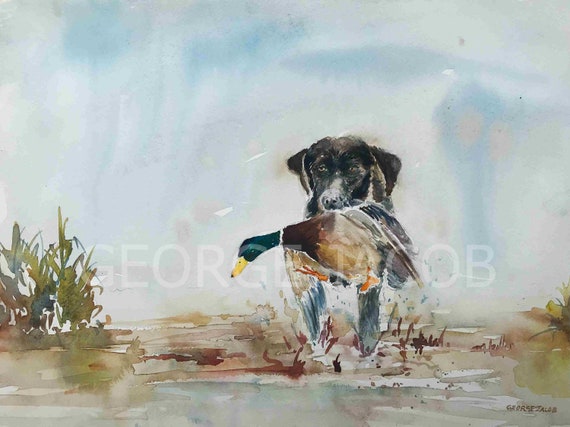The painting, likely a watercolor, depicts a black Labrador retriever with floppy ears and glistening fur, reflecting its wet condition. The dog is energetically splashing through a muddy, watery terrain, indicated by brown splashes surrounding its legs. Gripped firmly in its mouth is a vividly detailed mallard duck, identifiable by its green head, yellow bill, orange legs, and mix of brown and white feathers. The backdrop features a foggy, blue-gray sky, implying a misty atmosphere, with a hint of a pond or swamp landscape. Lush green vegetation, including reeds and moss, frames the lower corners of the image, adding depth to the scene. Two signatures mark the artist's identity: a semi-transparent white watermark reading "George Jacob" spans the whole painting, while a brown signature in the bottom right corner confirms the creator's name.